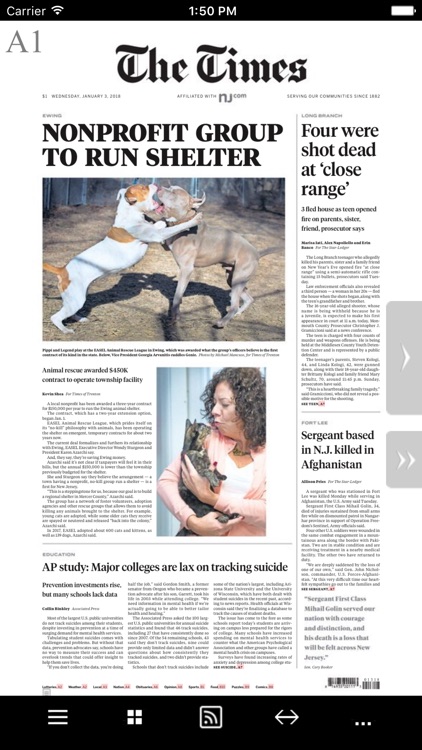This image is a screenshot taken from a cell phone displaying a webpage from the Times. In the top left corner of the screen, the "Carrier" label and the Wi-Fi symbol are visible. Centered at the top, the time is indicated as 1:50 PM. On the top right corner, the battery icon can be seen. Just below the "Carrier" label, there is a grayish 'A' and '1' in a large, capitalized font. Dominating the middle of the screen is the Times' distinctive, traditional black font logo.

Beneath the logo, the headline of the main news article reads, "Nonprofit Group Truron Shelter." The featured image under the headline shows two pit bulls that appear to be engaged in a fight. The dog on the left is predominantly white with brown markings, while the one on the right is a grayish color. Both pit bulls are standing on their hind legs with their mouths in close proximity, suggesting they might be biting each other.